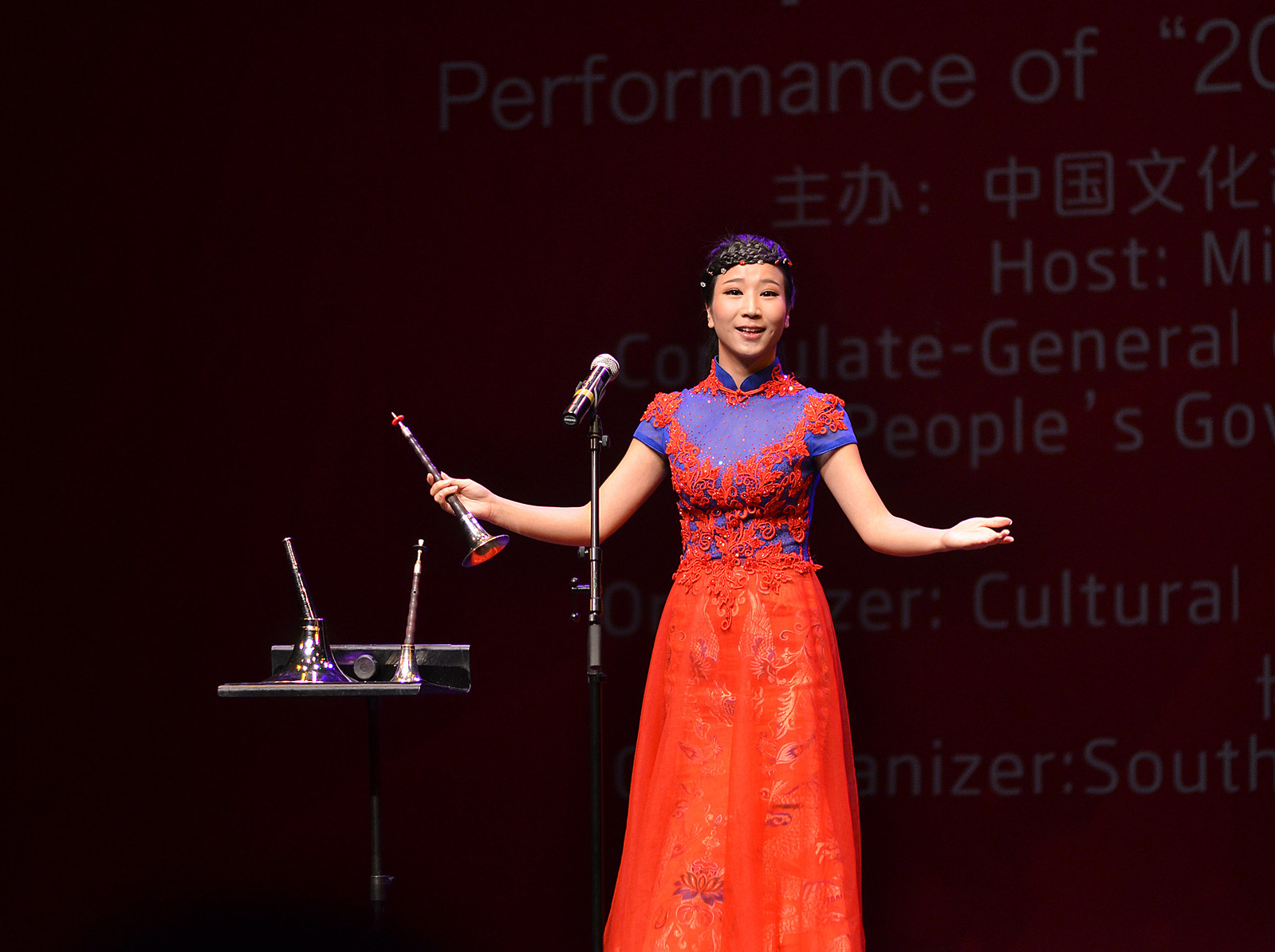In this wide rectangular photograph, a woman of Asian descent is captured mid-performance on a stage. She stands just to the right of the center, wearing a vibrant ensemble consisting of a long gown that transitions from bright blue at the top—adorned with intricate red-orange embroidery—to a vivid orange at the bottom. The gown appears to include transparent pants underneath. Her dark hair is sleekly pulled back, decorated with what seems to be purple jewelry or dyed accents.

The woman has white skin and is holding a small instrument resembling a horn, positioned at a microphone. To her right, the viewer's left, there are two additional horns on a stand. The backdrop features a faintly red-grayish shaded screen filled with white text and Chinese characters. Though partially obscured by the woman and shadows, the visible text includes phrases like "performance of," "consulate general," "people's," and "cultural." The far left side of the backdrop fades into darkness, creating a dramatic setting.